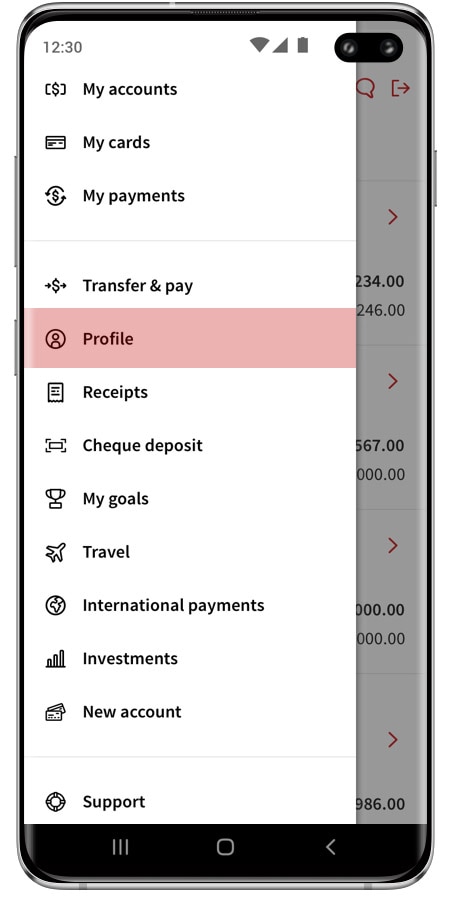The screenshot taken at 12:30 PM displays a phone with a full battery, active signal, and Wi-Fi connectivity. The phone features two forward-facing buttons, two buttons on the left side, a rocker button, a power button, and an additional button that resembles a power button. The interface suggests it might be an iPhone, given the overall design and button layout.

The screen showcases a menu related to financial management, set against a black text on a white background. The menu items listed include: My Accounts, My Cards, My Payments, Transfer and Pay, Profile (partially obscured by a pink bar), Receipts, Check Deposit, My Goals, Travel, International Payments, Investments, New Account, and Support. At the bottom of the screen, the typical navigation buttons - Menu, Home, and Back - are visible. 

In the background of the screen, there are indistinct numbers partially concealed by the overlaying menu, making them difficult to decipher. Overall, the display appears to be a financial management application with several comprehensive options for managing various financial tasks and accounts.